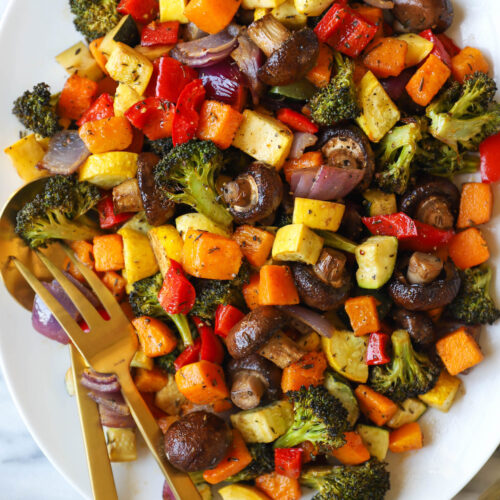This photograph showcases a vibrant and delicious-looking plate of roasted vegetables artfully arranged on a plain, round, white ceramic plate. The dish features an appetizing mix of broccoli, butternut squash, summer squash, zucchini, red bell peppers, whole button mushrooms, red onions, and possibly carrots, all glistening due to a light coating of olive oil or butter. The vegetables are seasoned with a modest sprinkling of herbs, like thyme or oregano, and freshly ground pepper, enhancing their natural flavors without overwhelming them. Two pieces of elegant gold silverware—a long, three-pronged fork and a partially hidden spoon—rest atop the colorful medley, adding a touch of sophistication. The photo is set against a white granite countertop, with the background subtly visible in the bottom left corner, highlighting the sheen of the plate and contrasting beautifully with the rich hues of the roasted vegetables.